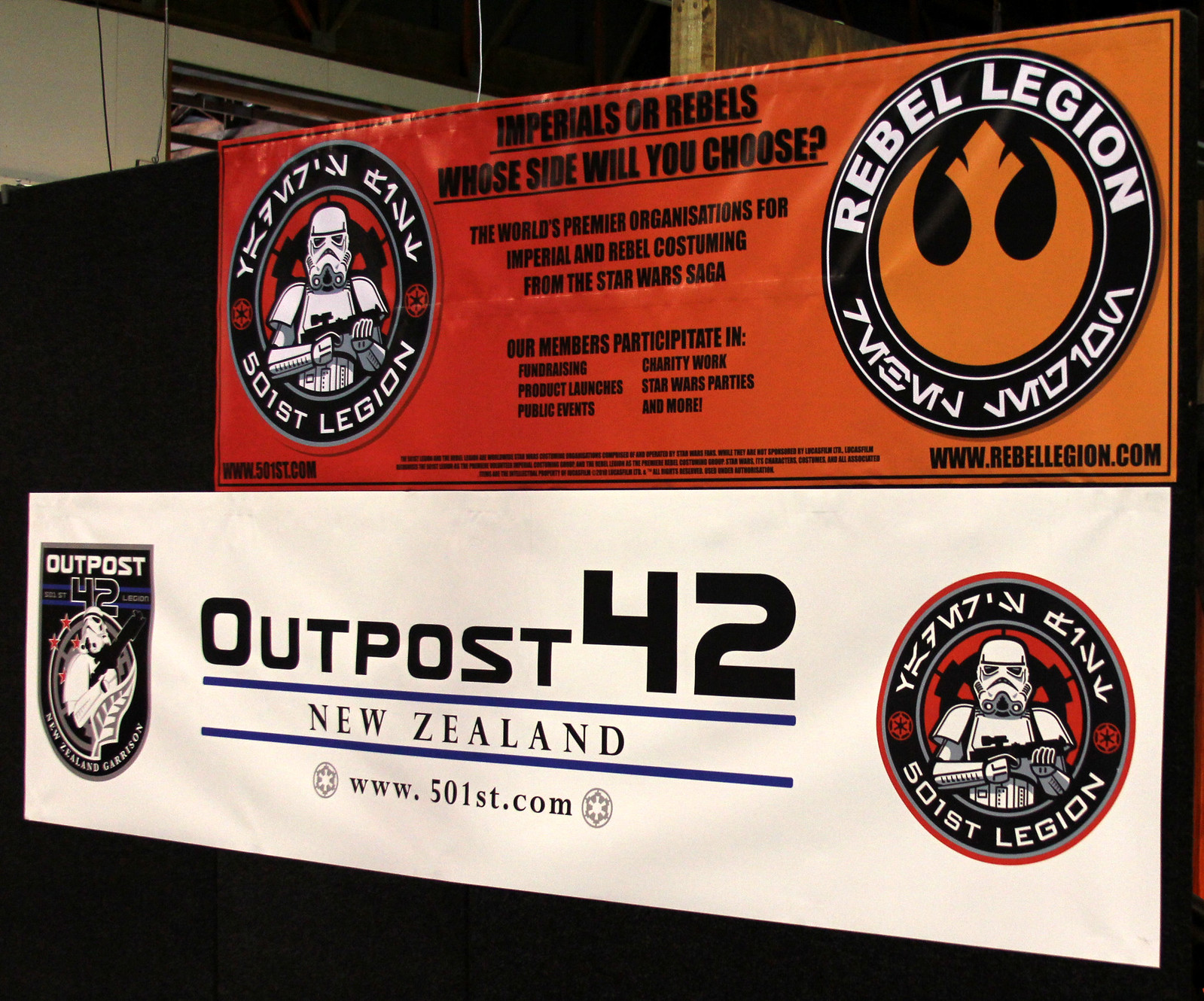This image, taken inside a building with a partial black wall, captures a display of two distinct banners, likely at a Star Wars convention in New Zealand. The top banner, set against a vibrant gradient of red to orange, prominently features the central question "Imperials or Rebels? Whose side will you choose?" accompanied by the logos and circular designs of the 501st Legion (with a stormtrooper) and the Rebel Legion. Surrounding the text are iconic Star Wars symbols and the phrase "The world's premier organizations for Imperial and Rebel costuming from the Star Wars saga." The lower right corner of this banner provides a URL: www.rebellegion.com.

Beneath this is a white, horizontally-aligned rectangular banner labeled "Outpost 42" with “New Zealand” below it. This banner features a prominent number "42" flanked by symbols and figures of stormtroopers, indicating its connection to the 501st Legion. Additional text includes "www.501st.com."

The overall scene suggests these signs are part of an informative display about Star Wars-related costuming organizations, specifically highlighting activities such as fundraising, public events, and charity work undertaken by members of these groups.